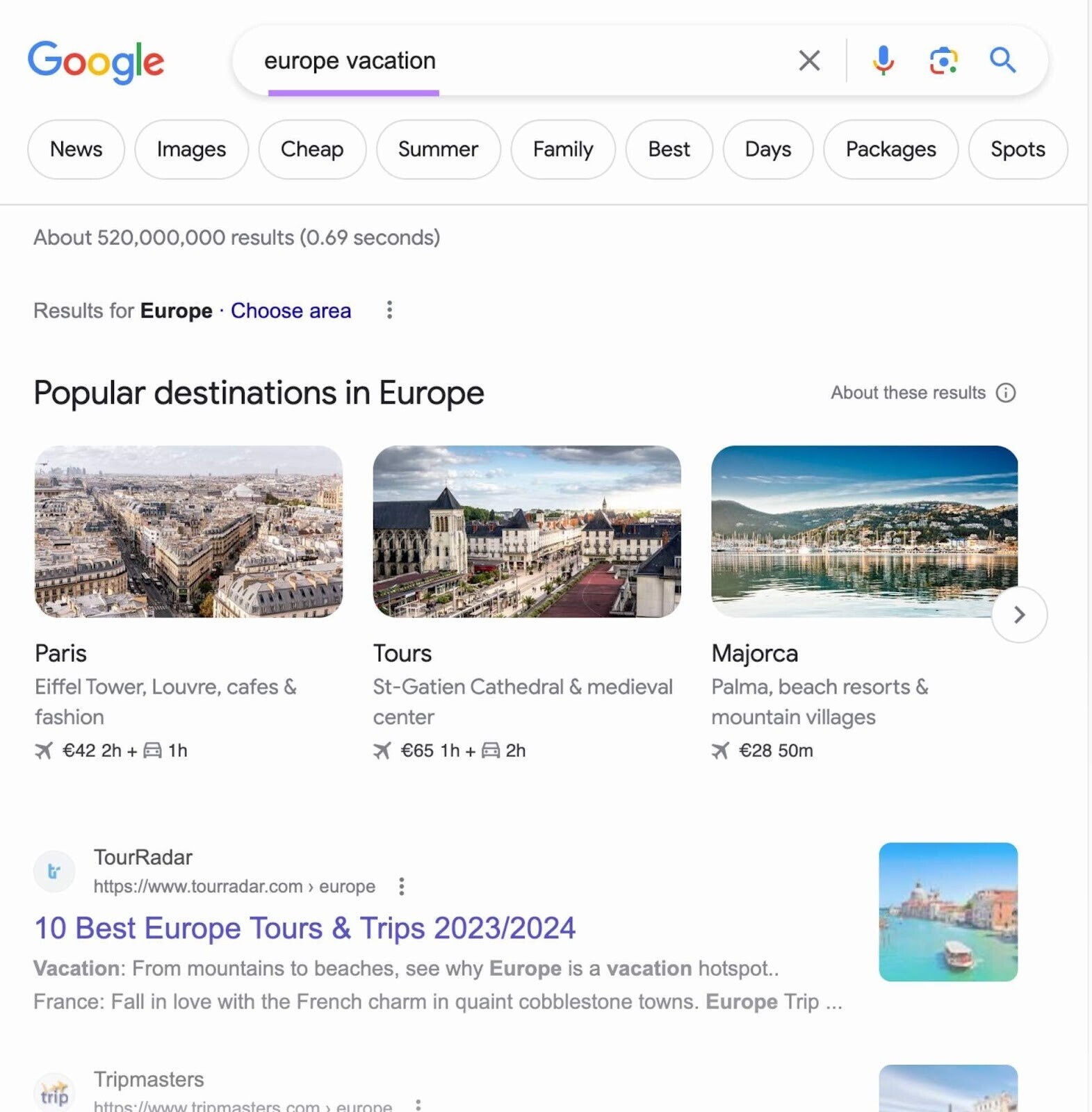Screenshot of a Google Search Page for "Europe Vacation"

The image is a vertical screenshot of a Google search results page for the query "Europe vacation." At the top left corner, the recognizable Google logo is displayed. Immediately to the right, a search bar featuring the text "Europe vacation" in black, with the text underlined in purple, is prominently positioned. The search bar is accompanied by several icons: a black X to clear the search, a blue and red microphone for voice search, an icon resembling a TV with a dot in the center likely representing Google Lens, and the traditional search magnifying glass.

Directly beneath the search bar, several category buttons are available for further filtering the search results. These buttons have a light gray outline with black text and include options like "news," "images," "cheap," "summer," "family," "best," "days," "packages," and "spots."

A light gray horizontal line separates the category buttons from the search results. The search results section begins with text indicating "About 50,520 million results (0.69 seconds)." It also includes a line stating "Results for" with "Europe" in bold and a blue link labeled "choose area."

Further down, in larger black font, the text "Popular destinations in Europe" introduces a series of three images showing different European travel destinations: Paris, Tours, and Majorca.